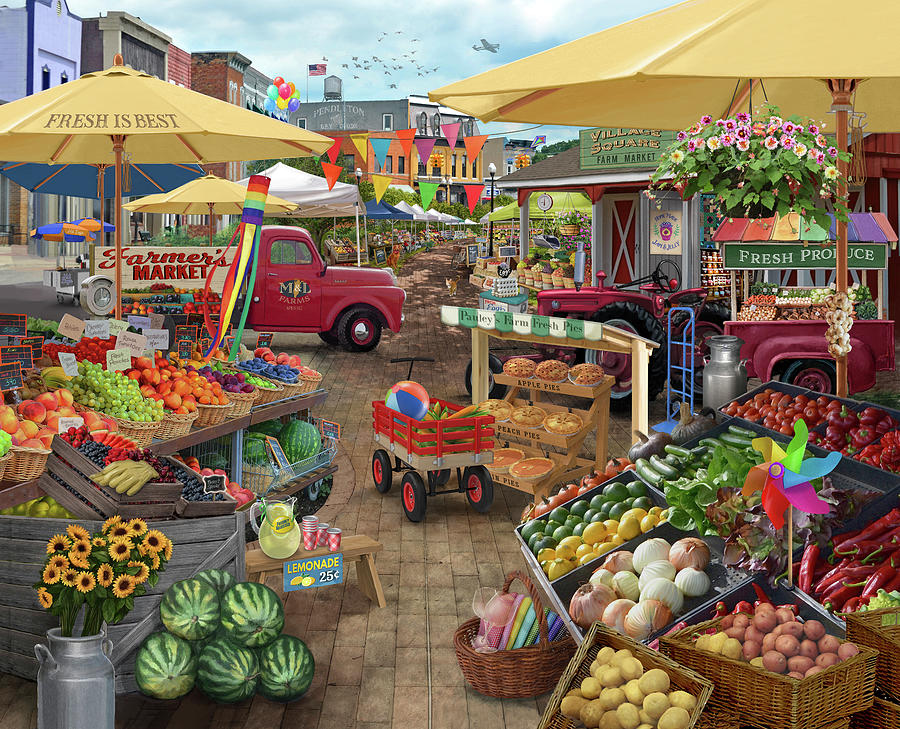This detailed digital image, seemingly a mix of lifelike and cartoonish elements, depicts an outdoor farmers market scene. The image is centered around two prominent market stands brimming with fresh produce, set against a bustling downtown backdrop. The stand on the left features wicker baskets filled with a variety of fruits such as peaches, grapes, plums, and blueberries, along with sunflowers in a bucket and a lemonade stand. A yellow umbrella with "Fresh is Best" printed on it and an old-timey red farmers' truck further define this stand’s charm.

On the right, another colorful stand showcases a plethora of vegetables including potatoes, red and brown onions, lemons, limes, zucchinis, tomatoes, and peppers. This stand is adorned with a rainbow-colored pinwheel and a flower basket alongside a sign reading "fresh produce." Between these stands, a smaller booth named "Polly's Farm Fresh Pies" offers apple, peach, and pumpkin pies. A red wagon filled with a beach ball and corn can also be seen in this vibrant scene.

The background features various buildings in hues of purple, brown, red, and gray with one prominently displaying the sign "Village Square Farm Market." An American flag waves atop, with birds and an airplane in the sky adding to the lively atmosphere. Balloons and more farm stands extend into the background under a cheerful triangle banner, emphasizing the market's bustling nature. The entire composition combines the realistic depiction of fruits and vegetables with a stylized, almost painted environment, creating a unique visual contrast that captures the viewer's attention.